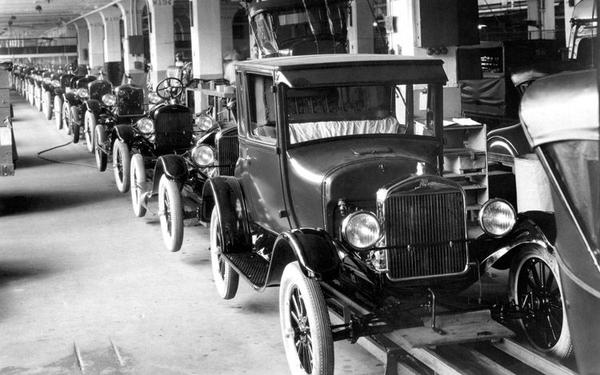The black and white photograph depicts an antique assembly line inside a car factory, likely from the early 20th century. The image, focused on a series of Ford Model T cars, extends into the background, creating a vanishing point that emphasizes the extensive scale of the production line. Each car, although incomplete, has already received its thin wheels and distinctive features such as large headlights, round taillights, and a square grille. The car nearest the camera appears nearly finished, sporting a hard, boxy top and exposed axles. Further down the line, vehicles are at various stages of assembly, notably missing their roofs but showing steering wheels pointing upwards. Rails beneath the cars indicate the tracks they follow along the concrete factory floor, where ropes or wires are visible. The factory workspace is expansive, with tall columns supporting the structure and a deck in the background, possibly for a foreman to oversee the operations. This detailed image evokes the industrious atmosphere of early automotive manufacturing.